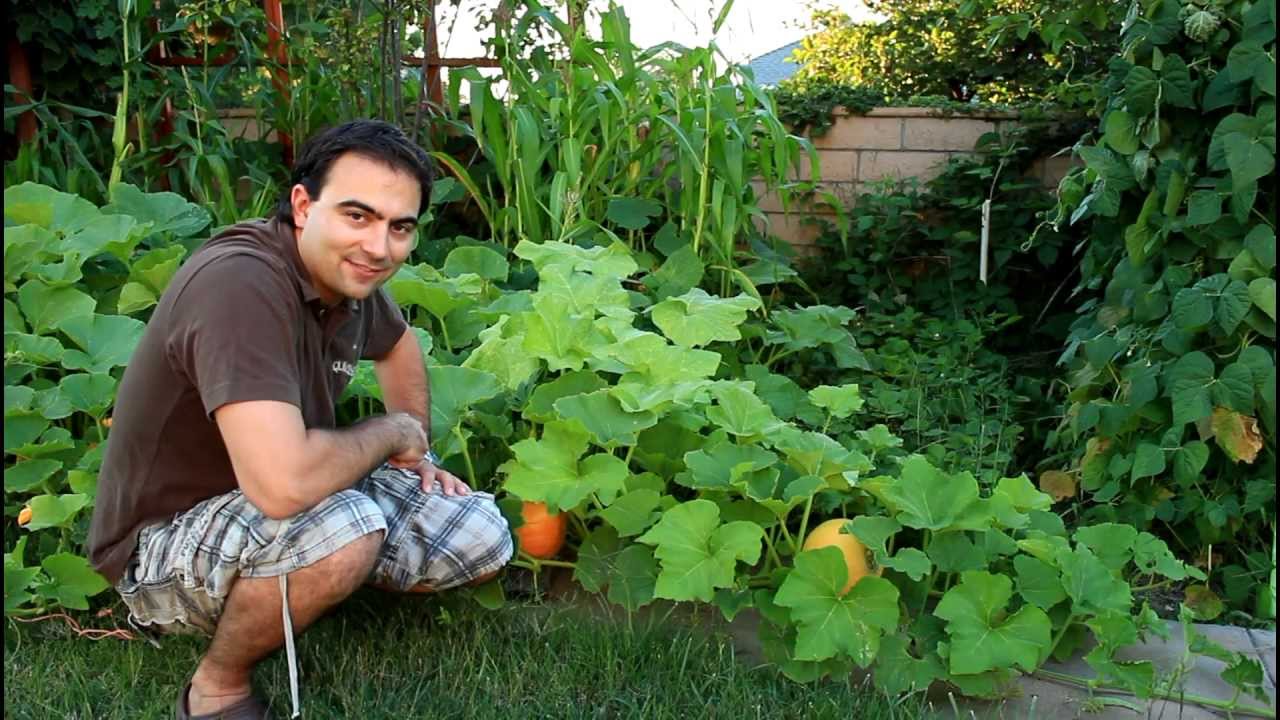A man, appearing to be in his 40s with dark hair and no facial hair, is featured in a lush garden. Positioned on the left side of the image, he is crouching or kneeling on green grass, with his right elbow resting on his right knee. He is dressed in a brown polo shirt and brown plaid shorts. Surrounding him is an abundant garden filled with leafy greens, amongst which various fruits and vegetables are partially visible. Bright orange pumpkins and buttery yellow squash, as well as other plants, can be seen peeking out from the foliage. To the left of the man, gourds and pumpkins are particularly noticeable. In the background, there's a low brick wall and an overgrown wooden ladder or trellis draped in vines, adding to the verdant setting. The man, deeply connected with his thriving garden, stands out against the vivid greenery.